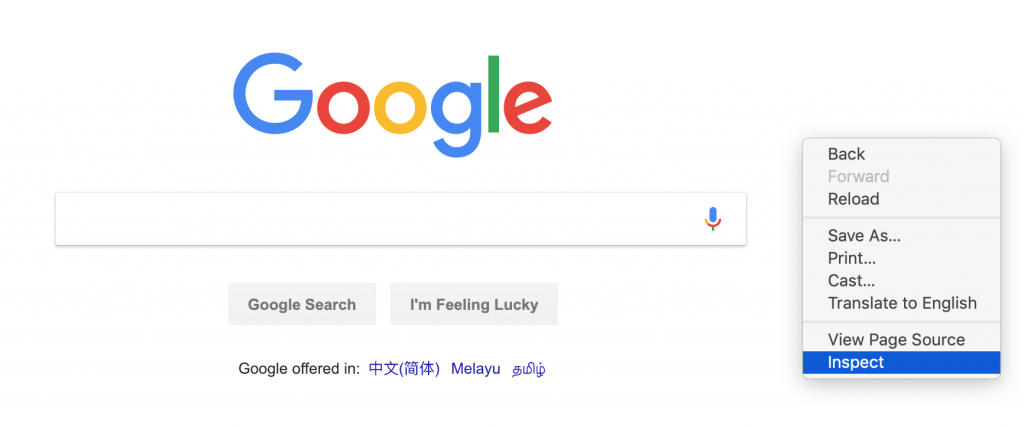This image is a cropped screenshot of the Google search page, viewed on a desktop computer. The top left of the screenshot showcases the prominent, large Google logo, centered at the upper section of the page. Directly beneath the logo is an expansive search box for entering queries, accompanied by a microphone icon on the extreme right for voice search functionality.

Below the search box, also centered, are two distinct gray buttons: the left button labeled "Google Search" and the right one labeled "I'm Feeling Lucky." Further down the page, centered text indicates language options, reading "Google offered in" followed by translations in Chinese characters, Malayu, and various Indian scripts.

On the right side of the page, there is an additional interface element—a context menu indicating a right-click action has been performed. This small gray box lists several options: "Back" at the top, "Forward," which is grayed out, followed by "Reload," "Save As," "Print," "Cast," "Translate to English," "View Page Source," and "Inspect." The "Inspect" option is highlighted, implying that the user has selected it.